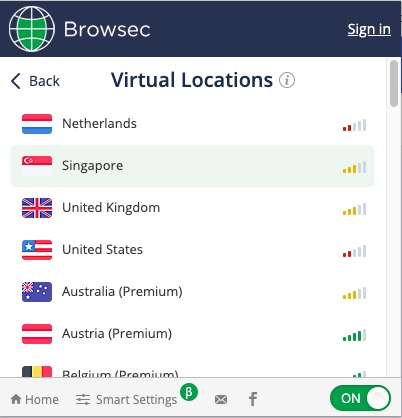The image is a screenshot of the Browsec website interface. The top section features a dark blue rectangle with the word "Browsec" displayed prominently in white text. To the left of the text is the Browsec icon, depicting a globe with latitude and longitude lines, rendered in white lines with green-filled sections within the globe. 

To the right of the Browsec name, the text "Sign In" appears in white. Below this header, the page displays the title "Virtual Locations" in black text. A list of countries follows, each accompanied by its national flag on the left side. The countries listed are: Netherlands, Singapore, United Kingdom, United States, Australia, Austria, and Belgium. 

Singapore is highlighted in a pale yellow-green color. Adjacent to each country name, there is a scale marked with five vertical bars, indicating connection quality or status. The specific markings for each country are:
- Netherlands: Two red bars at the lower end of the scale.
- Singapore: Three yellow bars.
- United Kingdom: Three yellow bars.
- United States: Two red bars.
- Australia: Three yellow bars.
- Austria: Four green bars.
- Belgium: Two green bars.